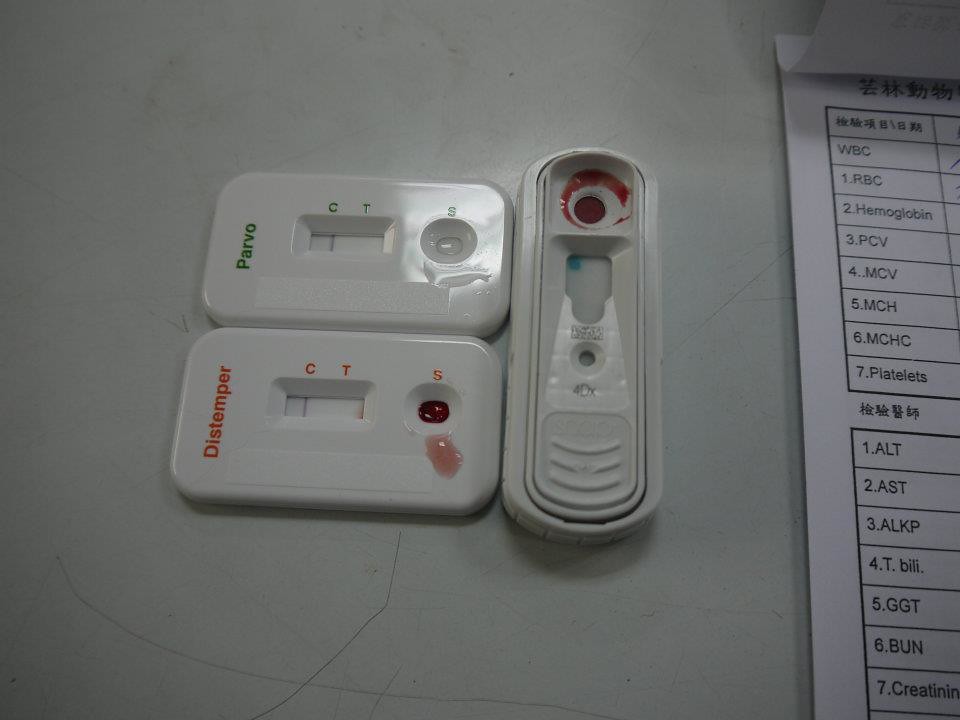The image, taken from a slightly elevated angle, depicts a medical setting, likely within a hospital or clinic. The focus is on a white countertop, which, despite its intended sterility, appears somewhat dirty and smudged, adorned with gray and black lines, especially concentrated towards the bottom and top regions.

On the far right of the countertop lies a stack of paper forms, designed so that individual sheets can be lifted to reveal additional layers beneath. The visible sheet on top features complex symbols from another language, arranged within numerous columns and rows. These columns list various blood work parameters, including WBC (white blood cells), RBC (red blood cells), hemoglobin, PCV, MCV, MCH, MCHC, and platelets, each represented by numerical data in sequences from one to seven.

Central to the page are blood sample results segmented into testing and control sections. These sections feature clearly labeled tests for parvo and distemper, along with a rectangular test strip adjacent to a differently shaped, oblong tester. The overall presentation suggests a comprehensive and systematic approach to blood analysis within a clinical environment.